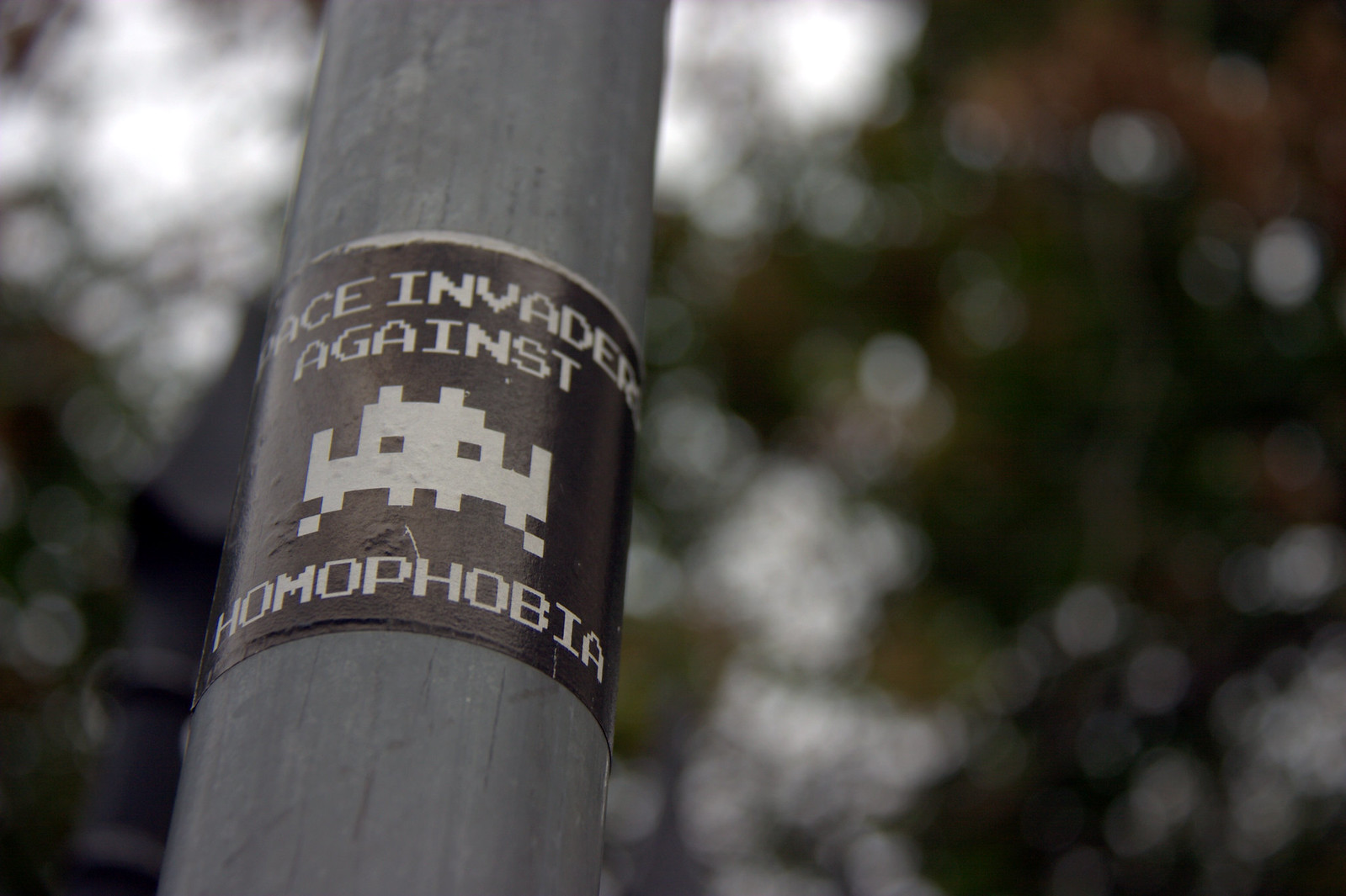This photo captures a grey metal pole, which serves as the main focal point. The shot is taken from a low angle, looking upwards, with blurred tree leaves and a hint of the sky in the background. Wrapped around the pole is a red sticker adorned with an 8-bit pixelated alien face reminiscent of Space Invaders. The sticker reads "Invaders Against Homophobia" in a retro video game font, with "Invaders" at the top, the alien face in the center, and "Against Homophobia" at the bottom. There are no other text or labels visible in the image.